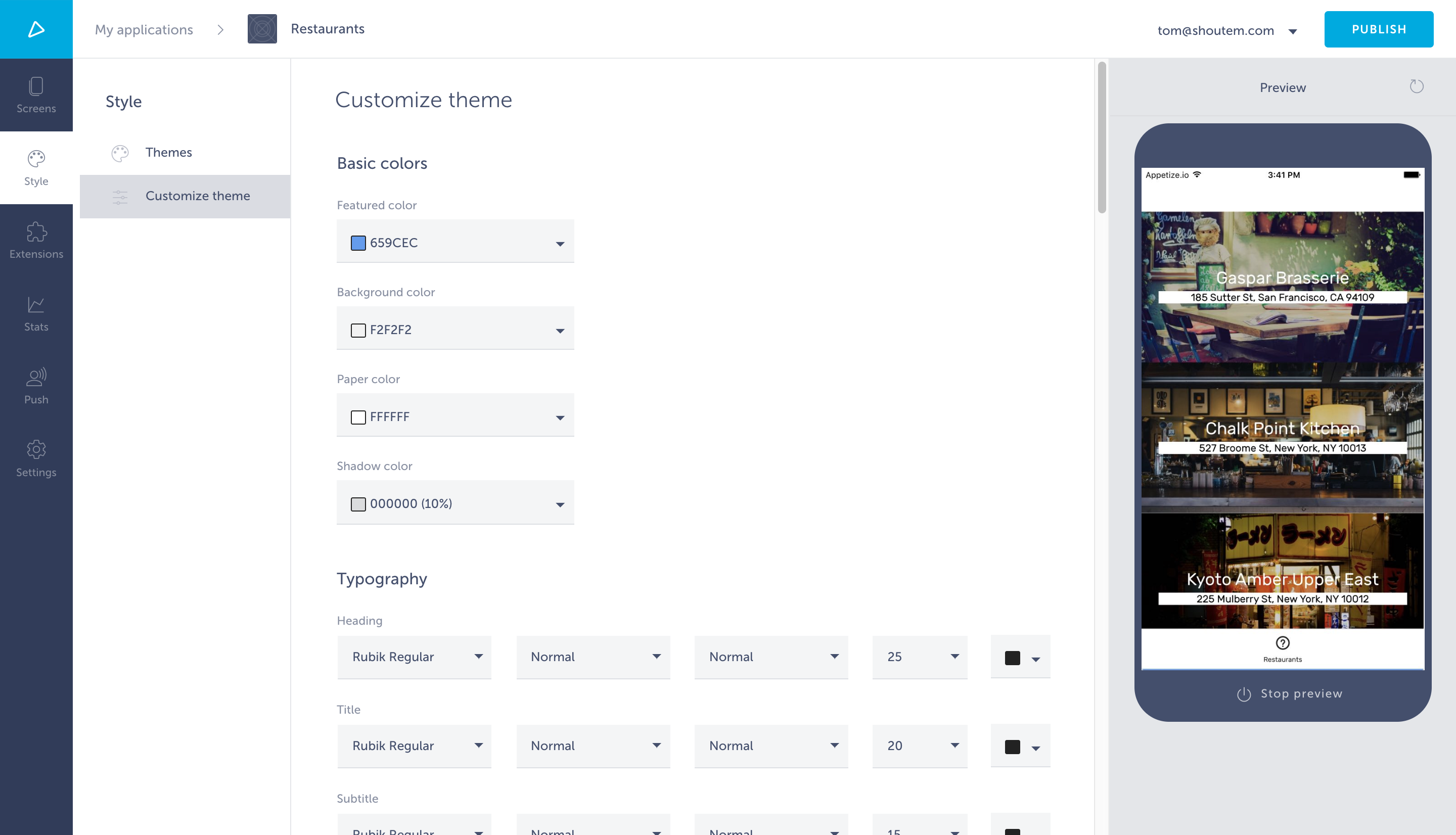This detailed and cleaned-up caption describes an interface for a restaurant website-building app:

---
A screenshot of a restaurant website-building app is displayed on a white background. On the right side of the screen, an iPhone mockup shows a live preview of a restaurant website template. The background of this preview pane is dark gray, highlighting the app's clean interface. On the left, a blue-colored sidebar is full of customizable options. Users can modify various attributes such as basic colors, typography, headings, and background colors from this menu. At the top of this sidebar, the app's name is displayed along with the text, "My Applications - Restaurants - Customized Theme." A prominent blue "Publish" button is also visible, ready for users to finalize and publish their custom restaurant website.

---

This caption gives a comprehensive description of the image, focusing on both the design and functionality of the app interface.